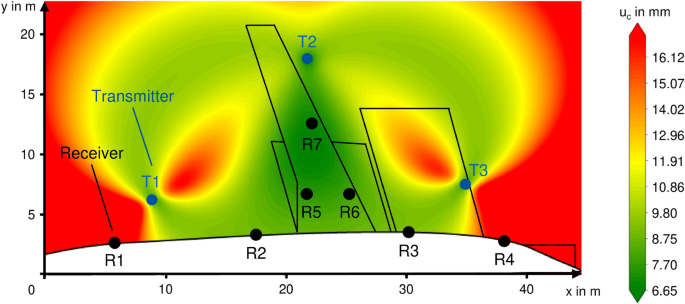This image depicts a detailed infrared graph with multicolored heat signatures representing various metrics. At the core, the graph displays contrasting colors—dark red to bright yellow to dark green—likely indicating temperature variations. The left axis, labeled "YNM," is numbered from 0 to 20, while the bottom axis—marked as "XNM"—ranges from 0 to 40. Embedded within the colored sections, terms like "transmitter" and "receiver" are prominently featured. The graph also includes numerous data points labeled R1 through R7 and T1 through T3, which appear to denote specific readings or components within the image. Additional annotations such as "UC" with a subscript "c" and measurements in millimeters (mm) are present, alongside numerical specifics like 6.65, 16.12, and others. The graph effectively conveys complex data through its vivid and structured layout.